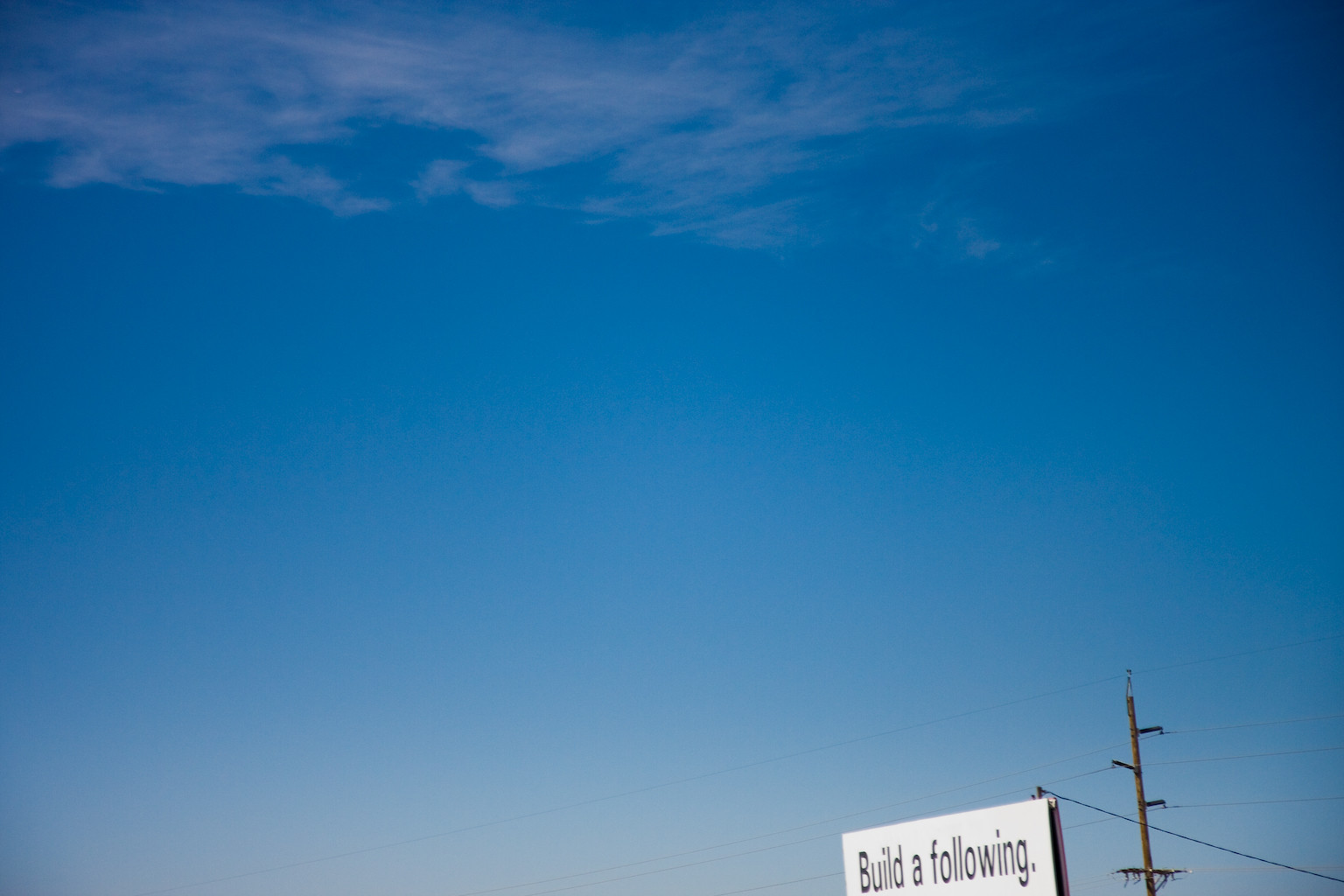This outdoor photograph, taken on a mostly clear day, features a captivating blue sky with varying shades; it's darkest in the center and upper-right corner, and slightly paler at the bottom. Wispy clouds are scattered across the top of the image, adding depth and texture. The photo is rectangular with a landscape orientation, showcasing a slice of the sky's vastness. In the lower right corner, partially visible, is a billboard featuring a white rectangular sign with black lettering that reads "Build a following," though the text below is cut off. Adjacent to the billboard is an electrical power line pole, with faint wires stretching across the lower part of the image from left to right.